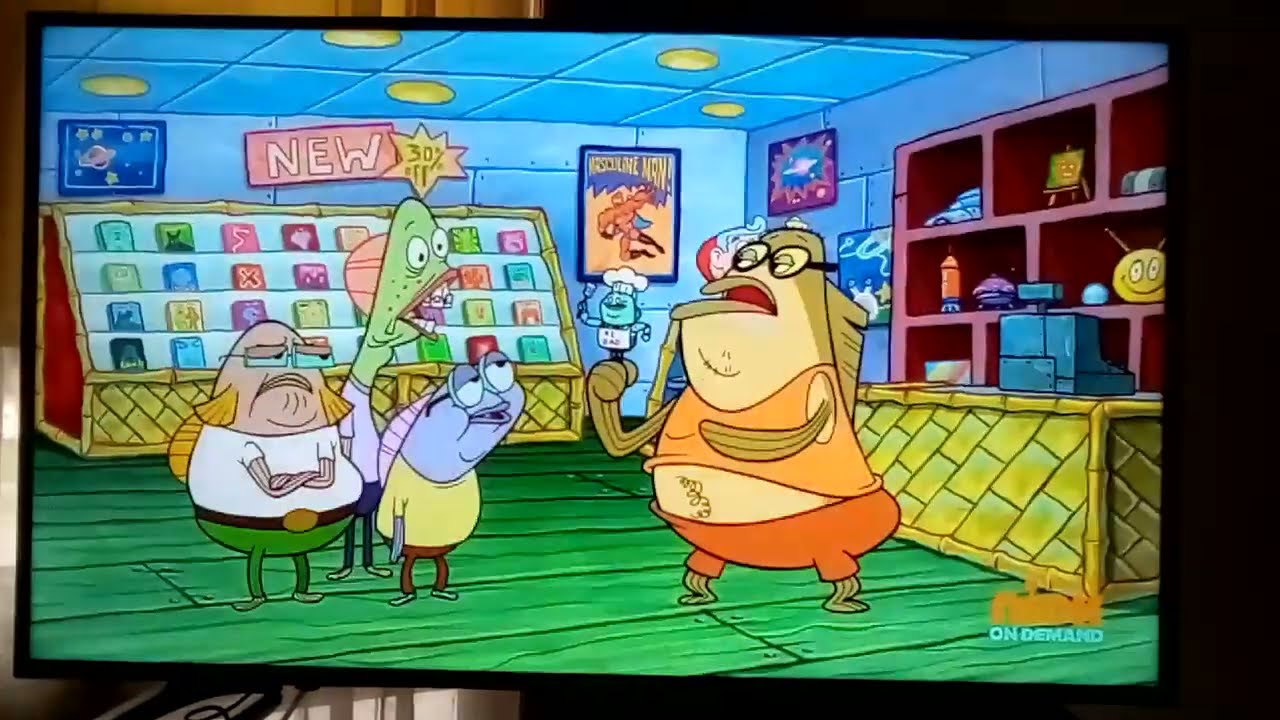In this vibrant cartoon image, seemingly a scene from the SpongeBob SquarePants show, we are transported to an underwater store adorned with whimsical details. The shop, glowing under yellow globe lights from the blue ceiling, features various shelves and stands filled with colorful items and albums. The backdrop includes a selection of CDs or DVDs, while the back wall is decorated with an image of stars and planets, giving it a cosmic ambiance. A prominent pink sign reads "NEW" and a yellow "30% OFF SALE" sign adds to the lively atmosphere. A bright yellow counter with a gray cash register sits to the right, flanked by shelves displaying an assortment of cartoonish doodads, including an easel, a small car, rocket, spaceship, and a smiley face. Central to this bustling scene are four cartoon fish characters, each with distinct appearances and expressions; one fish is holding a microphone-like object while the others look on, displaying a range of emotions from grumpy to droopy. This eclectic group of fish stands in a unique shop, blending the mundane with the fantastical in true SpongeBob fashion.